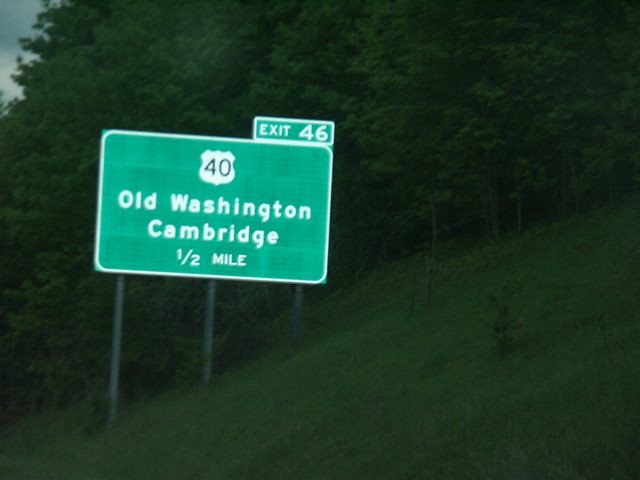In this detailed image, a highway sign stands prominently, informing drivers of upcoming destinations. At the base, a gently sloping landscape of green grass sets the scene. The sign is supported by three metallic gray poles of varying heights: the tallest on the left, a medium-length one in the center, and the shortest on the right. The sign itself has a green background and is square-shaped. At the top in bold black text, it displays the number "40." Directly beneath this, in white text, it reads "Old Washington, Cambridge, ½ mile." Additionally, there is a smaller rectangular sign mounted on the top right of the main sign, indicating "Exit 46." The backdrop features green trees, creating a lush, natural setting, with a patch of open, gray sky visible in the top left corner.